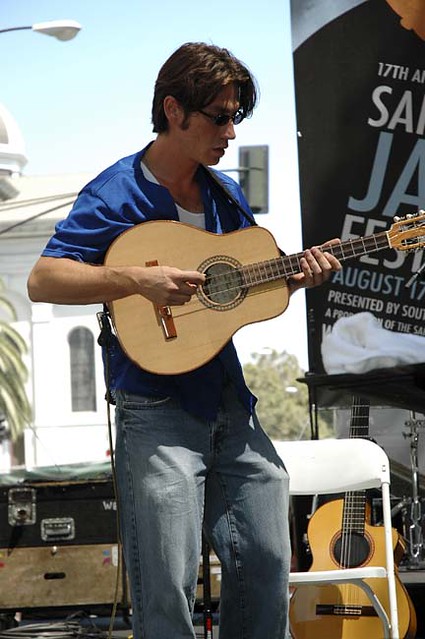In the image, a male musician aged around 30 to 40 years is captured passionately playing an acoustic guitar at an outdoor event. He stands against a bright, sunny backdrop that reveals a clear, cloudless sky. He is dressed in baggy blue jeans and a medium blue shirt with a white tank top underneath. His shaggy brown hair and dark-colored glasses add to his casual, yet focused demeanor.

The setting appears to be a stage in front of a large white government building, possibly a city hall with a dome reminiscent of the US Capitol. This governmental building and nearby trees create a picturesque backdrop. Visible equipment includes another guitar and a drum set, suggesting a well-prepared musical stage. 

In the background, a sign with a black background and white lettering reads "17th Annual SA," with large blue letters "JA" prominently visible beneath. This indicates the event is likely the annual jazz festival held on August 17th. The scene, filled with the sounds of music and an enthusiastic atmosphere, perfectly captures a vibrant moment during the festival.